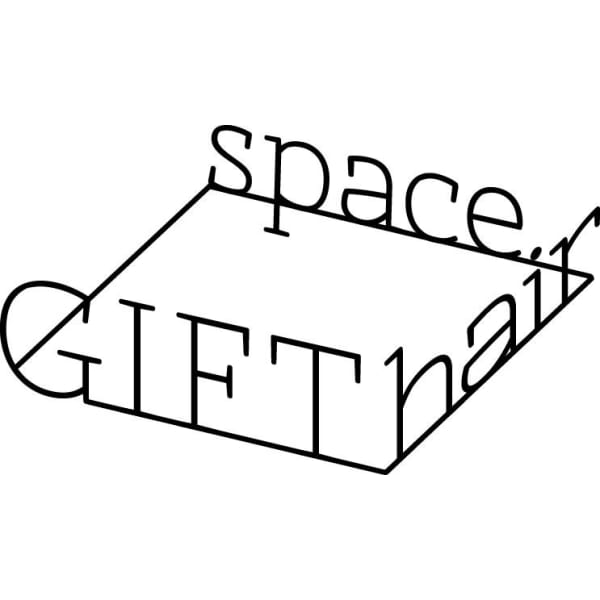This black and white image features a 3D art illusion using text. The primary element is a rectangle (or square, appearing rhombus-shaped due to perspective), tilted at an angle with an empty center. Three sides of this shape have words printed in black, creating the appearance of three walls in a mind-bending style. The top edge has the word "SPACE" standing along it, the right edge has the word "HAIR," and the bottom edge has the word "GIFT," all aligned with the borders of the shape. The left edge remains empty. The overall design plays with perspective, engaging viewers to perceive depth and dimension in the simplistic, monochromatic layout.